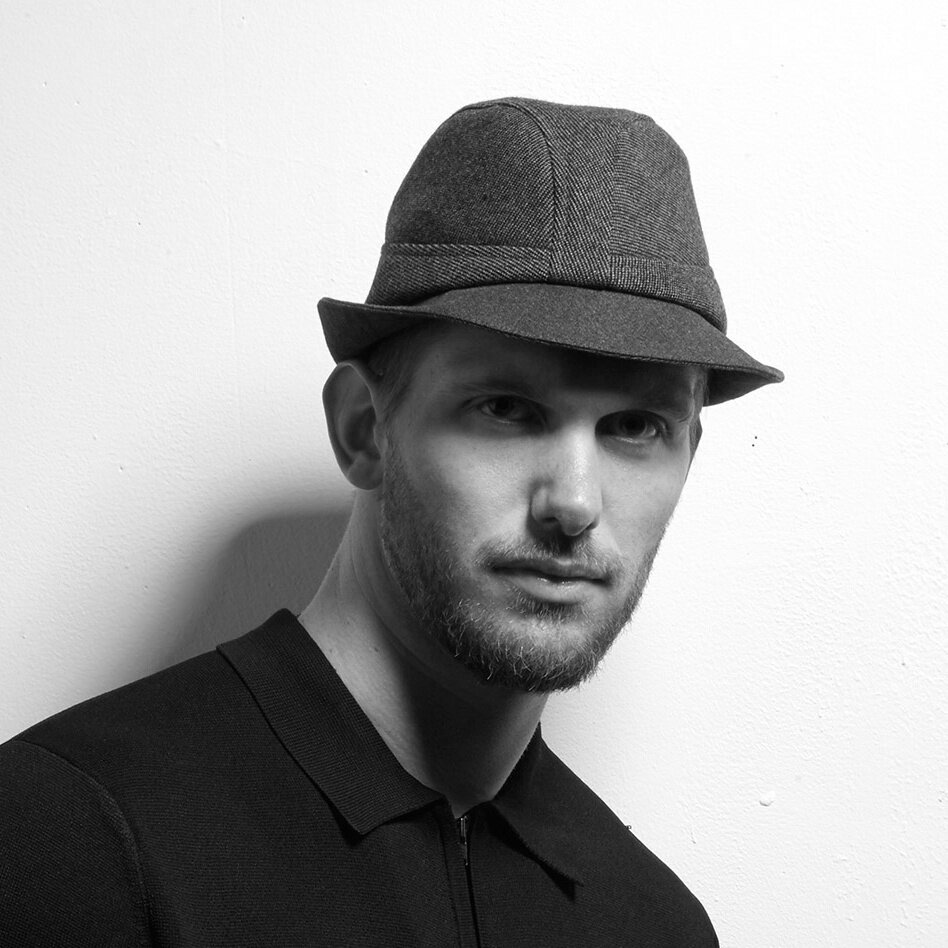This black and white photograph depicts a young Caucasian man, possibly in his mid-twenties, positioned against a whitewashed wall. He is wearing a dark, tweed cap with a small brim that casts a shadow over his eyes, making their color indiscernible. His facial expression is serious, and he has a light, scruffy beard — with the stubble being lighter on the cheeks and fuller around his chin and mustache. He’s dressed in a black polo shirt or light jacket with a zipper running up to the collar, and the photograph captures him from the shoulders up. Although most of his hair is hidden under the cap, some short-cut hair is visible above his ears. His head is slightly cocked, showing only one ear prominently, and his full lips and prominent nose are clearly defined.